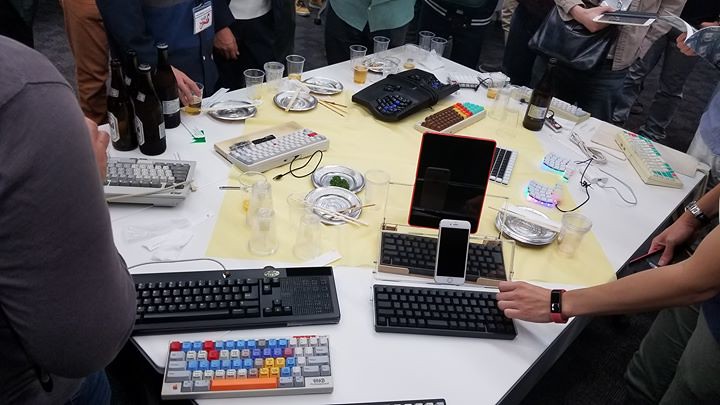This image depicts a bustling conference or event centered around a large, white, rectangular table partially covered by a square cloth. Scattered across the table are about eight mechanical keyboards of various colors, shapes, and sizes, including a unique one with keys that resemble hamburger ingredients. The keyboards are accompanied by several electronic devices, including iPhones and iPads, likely connected via Bluetooth or Wi-Fi. In addition to the tech gadgets, the table hosts an assortment of items such as four black beer bottles, several clear plastic cups filled with a brown liquid, a wine bottle, and multiple empty plates and glasses. Surrounding the table are the torsos of six to eight people, possibly holding pamphlets, all engaged with the devices and keyboards. The scene suggests a hands-on workshop or tech meetup, where participants are deeply involved in exploring and experimenting with various electronic devices.